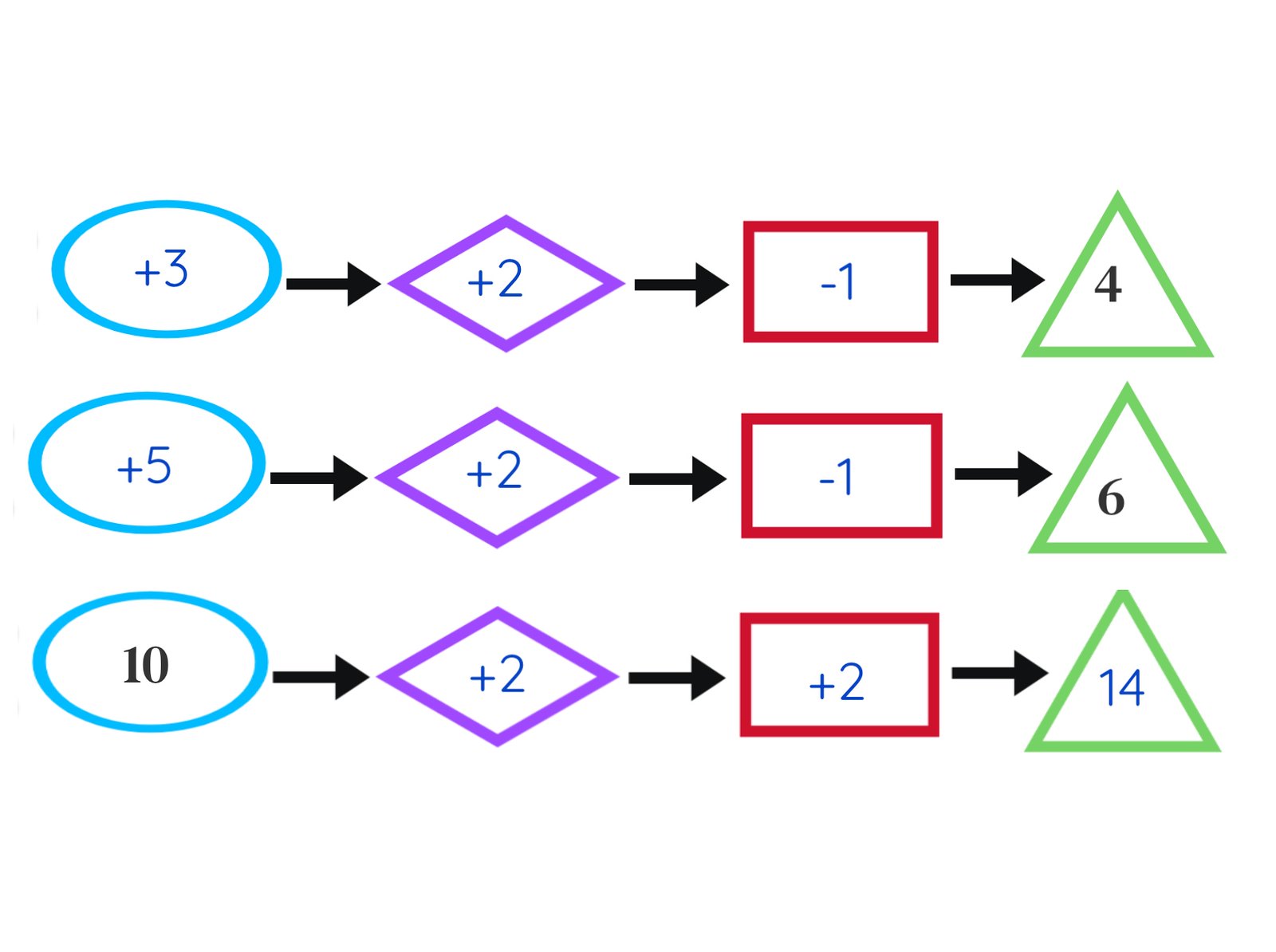Here is the cleaned-up and detailed caption:

The image depicts a sequence of columns made up of various geometric shapes and numbers arranged in three rows. Starting from the leftmost column, we have a column of ovals. In the first row, the ovals contain the numbers +3, +2, and -1. Moving down to the second row, the ovals display +5, +2, and -1. In the third row, the numbers within the ovals are 10, +2, and +2.

To the right of this column is a column comprised of black arrows pointing to the right.

Following this is a column of purple diamond shapes. The numbers within these diamonds, from top to bottom, are 4 in the first row, 6 in the second row, and 14 in the third row.

Next to the column of purple diamonds is another column of black arrows pointing to the right.

Continuing to the right, there is a column of red rectangles. These rectangles contain unidentified numbers.

Another column of black arrows pointing to the right follows the red rectangles.

Finally, the last column is made up of green triangles, each containing an unspecified number.

The arrangement and numeric pattern within the shapes seem to follow a specific sequence or logic that might be significant to the overall image.